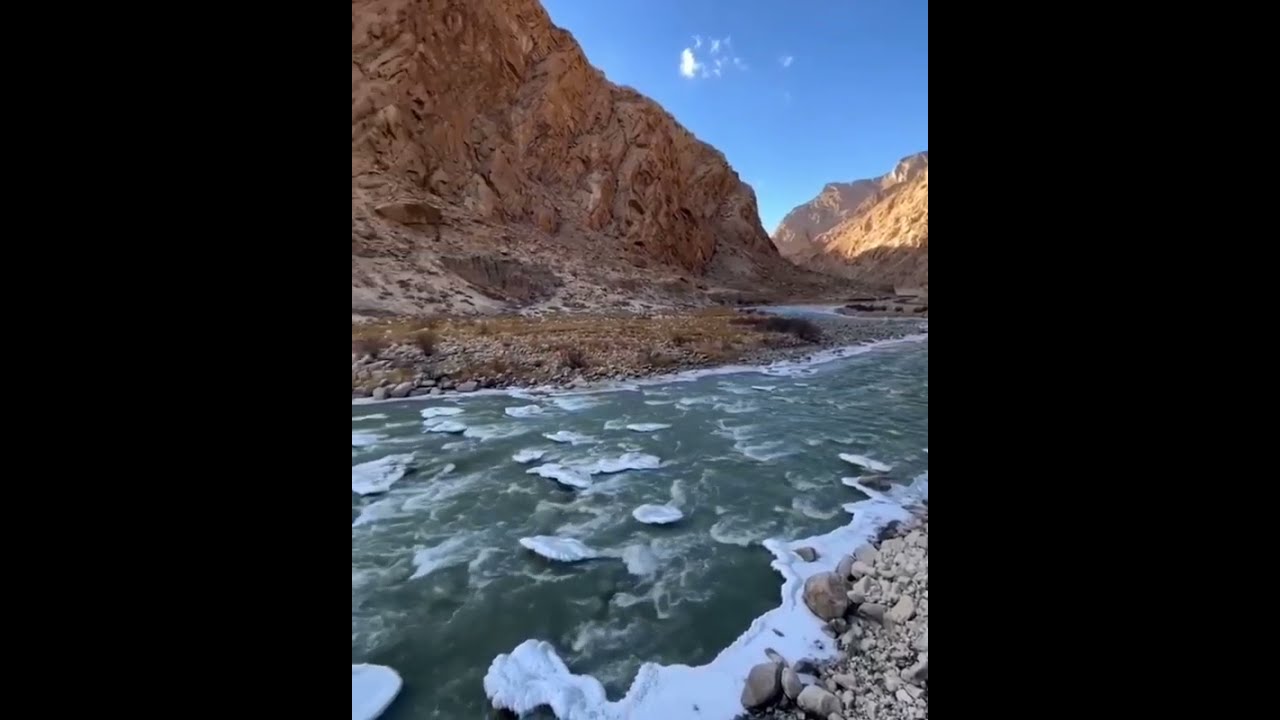The image captures a bright, sunny day along a fast-running, shallow river flanked by rugged, low-lying cliffs within a desert canyon. The river, about a dozen meters across, features choppy, white-capped rapids that give the water a bluish-gray hue, contrasting with the sunlit and shaded rocky terrain on either side. Various stones break through the surface, indicating the river's shallowness, while patches of snow and ice along the banks suggest a cold temperature despite the clear blue sky. The surrounding landscape is arid and predominantly rocky, with minimal vegetation, evoking a serene yet rugged environment that's perfect for a scenic walk.